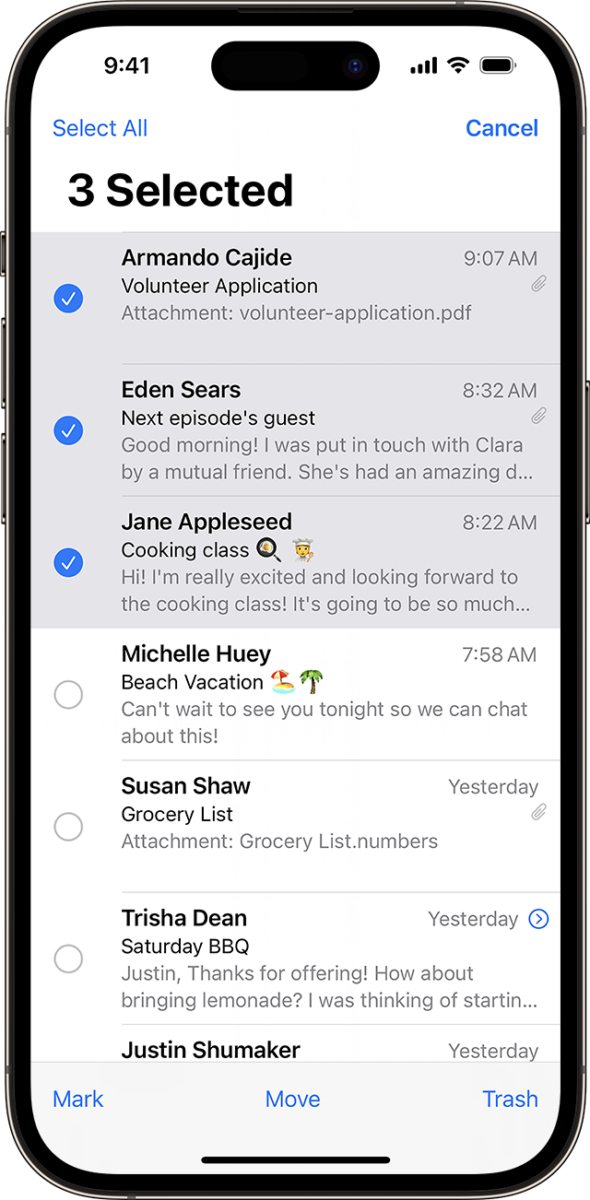This is an image of a smartphone screen displaying an email application. The smartphone itself features a black border. The screenshot captures the “Main Screen,” with the section heading labeled as "Three Selected." At the top, there is a header bar that includes a link labeled "Select All" in blue, a "Cancel" link, the current time, and icons for Wi-Fi signal strength and battery level.

The screen shows a list of emails, with the first three emails highlighted with a light gray background and a blue check mark in a circle to the left, indicating they are selected. These emails also display the sender's name and subject line. The first email is from Armando Kahide with the subject "Volunteer Application," the second is from Eden Sears titled "Next Episode's Guest," and the third is from Jane Appleseed with the subject "Cooking Class." Both the first and second emails have a paper clip icon underneath the time, suggesting the presence of attachments.

The subsequent three emails are not selected and display a white background. The fourth email is from Michelle Huey titled "Beach Vacation," followed by an email from Susan Shaw with the subject "Grocery List," and an email from Tricia Dean about a "Saturday Barbecue." The final email shown is from Justin Shoemaker, though the subject is partially obscured by the bottom menu bar.

At the bottom of the screen, there are three clickable blue icons labeled "Mark," "Move," and "Trash," offering different actions for the selected emails. The interface design and arrangement of elements provide a clear and concise user experience for handling emails on the smartphone.